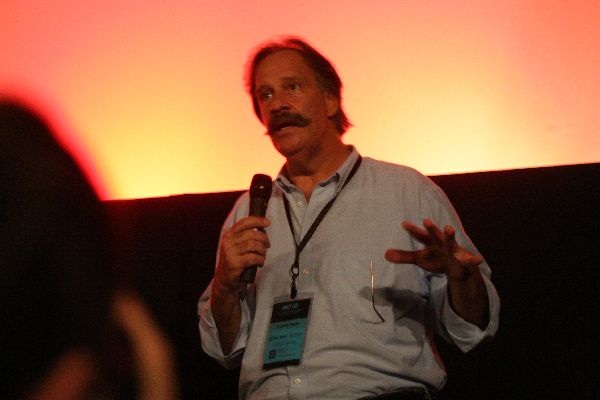A man stands on stage, mid-speech, with a lanyard bearing a card around his neck. He holds a black microphone in his right hand while his left hand is extended, palm facing down with fingers spread. He sports a thick, bushy mustache, brown eyebrows, and his hair is slightly receding. His button-up shirt is blue-gray, adorned with white buttons, and the sleeves are neatly rolled up to his elbows. Hanging from his shirt pocket are glasses. The background features out-of-focus lights with a yellow and pink hue, creating a sunburst or fire-like effect. The partial outline of an audience member's head is visible in the bottom left corner.